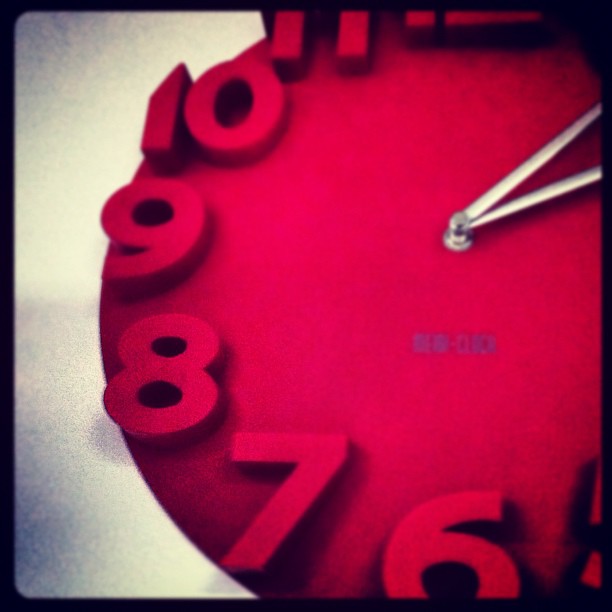The image is a close-up of a circular, bright pink clock with white hands, set against a grayish-white background. The clock face is designed to look like a flat pink disk with large, three-dimensional numeric digits positioned around the outer edge. However, the digits are somewhat out of scale for the clock's size. The visible numbers range from 6 to 12, though parts of 5, 11, and 12 are slightly cut off, and the numbers 1 to 4 are completely hidden. Beneath the clock hands, which are centered but extend out of frame, there are small blue symbols—possibly Chinese or Japanese characters. The clock face lacks a protective glass covering. The entire picture is framed with a black border with curved corners. There are sporadic dark spots on the wall in the background, adding a subtle texture to the backdrop.